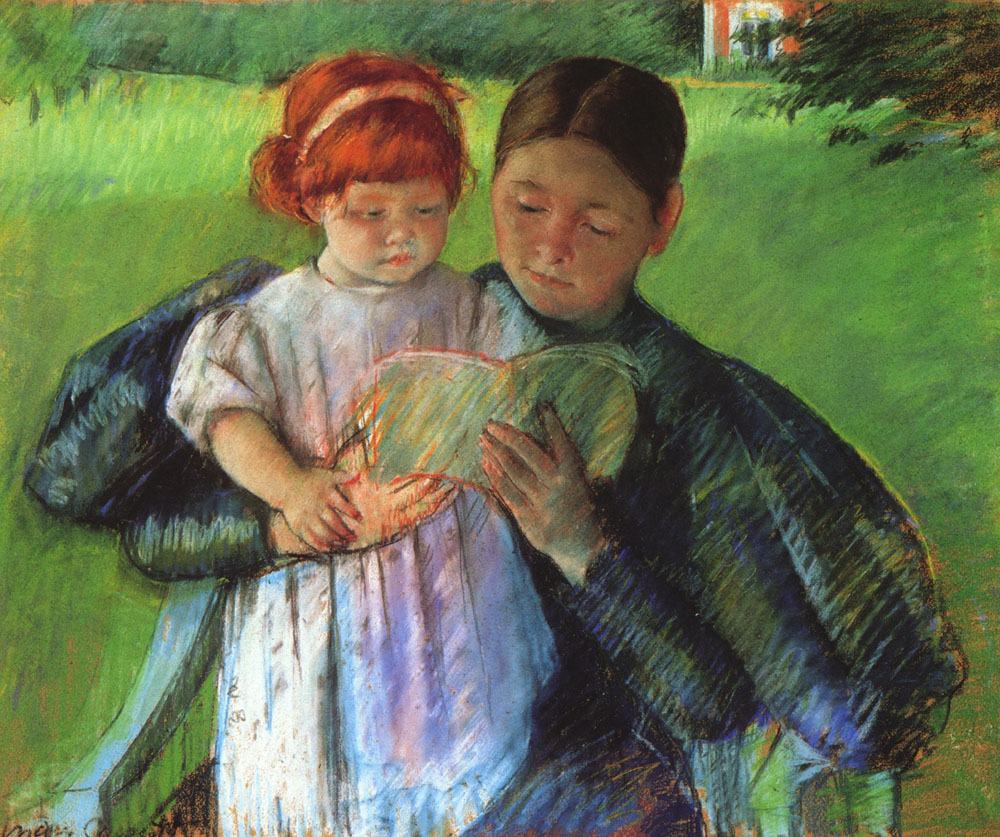This photograph captures a detailed painting of a serene garden scene from the 1800s. At the center, a young woman with neatly combed brown hair sits on a blue and white chair with a brown cushion, reading to a small child perched on her lap. The woman wears a traditional, long-sleeved, blue dress with large, poofy sleeves, and she holds a green-covered book in her left hand while her right arm gently supports the child. The child, around 4 or 5 years old, has bright red hair adorned with a pink headband and wears a short-sleeved, white dress. Both are intently focused on the book. In the background, a lush garden brimming with trees and plants creates a picturesque setting, with a red brick house featuring a white-edged corner and a white framed window peeking from the top right corner.